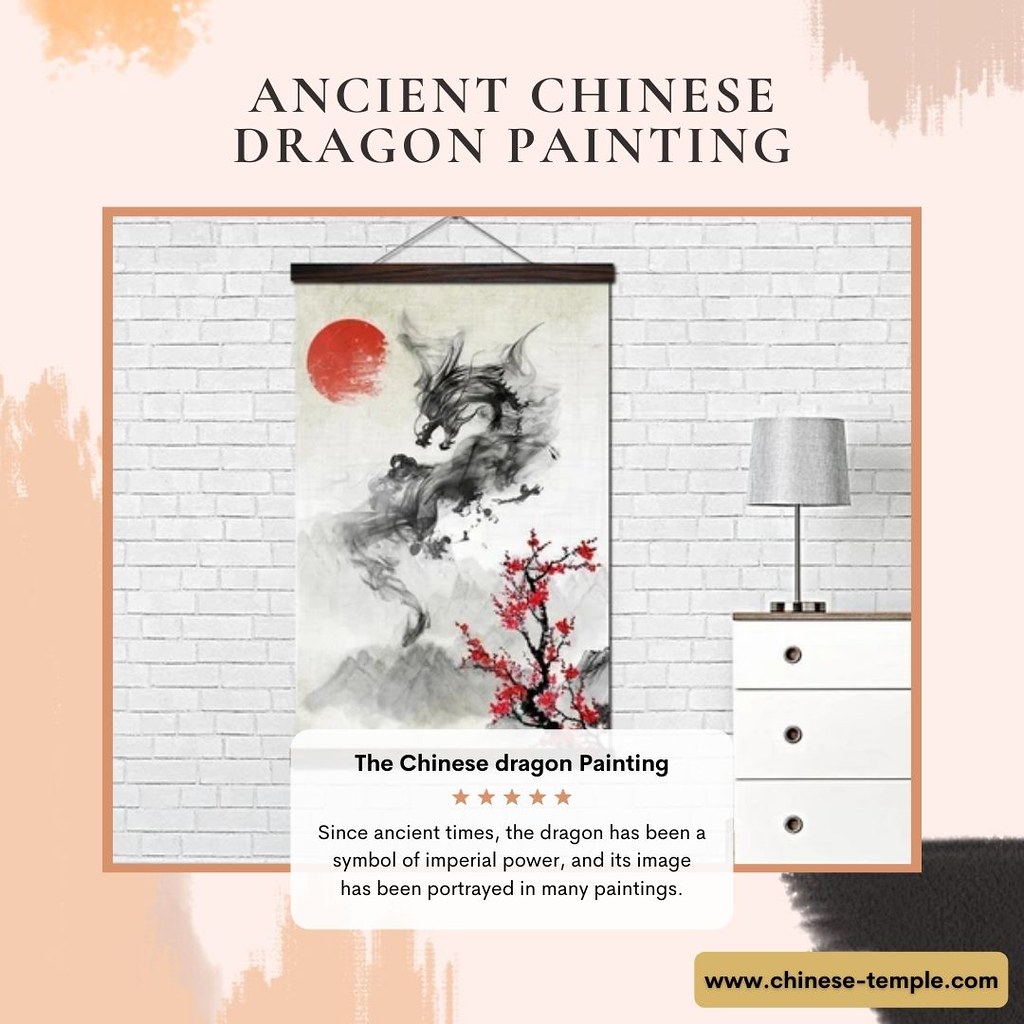The image depicts an advertisement for an artwork described as an "Ancient Chinese Dragon Painting" in prominent black lettering at the top center. The background is primarily a peach color with varying splotches of darker peach. The centerpiece of the image features a white brick wall upon which a traditional scroll painting hangs. This painting showcases a dragon rendered in a smoky black design, accompanied by a red moon located in the upper left corner and a depiction of what appears to be red cherry blossoms or flowers in the bottom right. Additionally, grey mountains are subtly illustrated below the dragon. Adjacent to the artwork, a white wooden dresser with a gray lamp is visible, positioned against the white brick wall. Enhanced by five gold stars, the description beneath the painting reads: "Since ancient times, the dragon has been the symbol of imperial power and its image has been portrayed in many paintings." At the bottom right of the image, the website www.chinese-temple.com is listed.